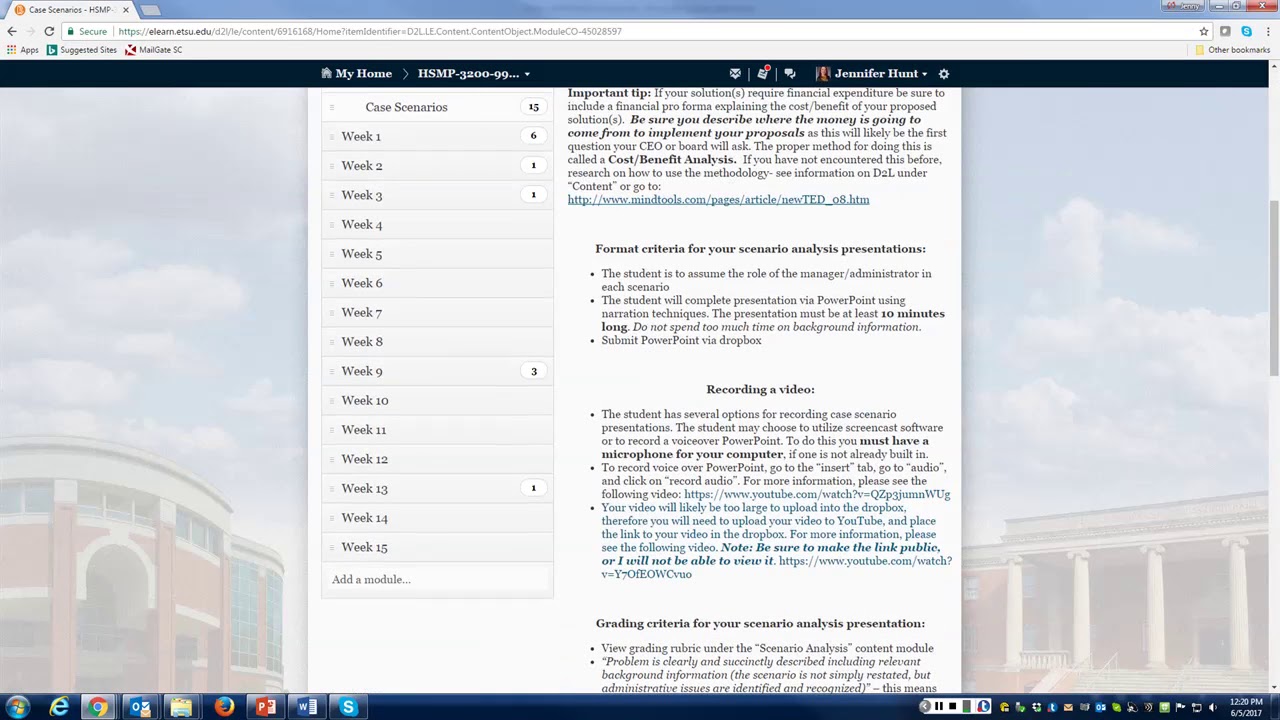The image depicts a webpage with suboptimal quality, appearing blurry, fuzzy, and pixelated. Despite the poor resolution, some elements can still be discerned. At the top left corner, the browser tab is labeled "Case Scenarios, HSP, HSMP." Directly below the tab, navigation buttons for "Back," "Forward," and "Refresh" are visible, followed by a search bar on the right, though the URL in the search bar is illegible due to the size and blurriness of the text. 

In the top left of the webpage interface, there are standard window control buttons for minimizing, maximizing, and closing the window. The webpage is divided into two main sections. The left section features a list labeled "Case Study" at the top, with entries for each week from Week 1 through Week 15 arranged vertically. The right section contains a text block titled "Important Tip," offering advice related to financial expenditures associated with the case study solutions, though the exact phrasing is unclear due to the image quality.